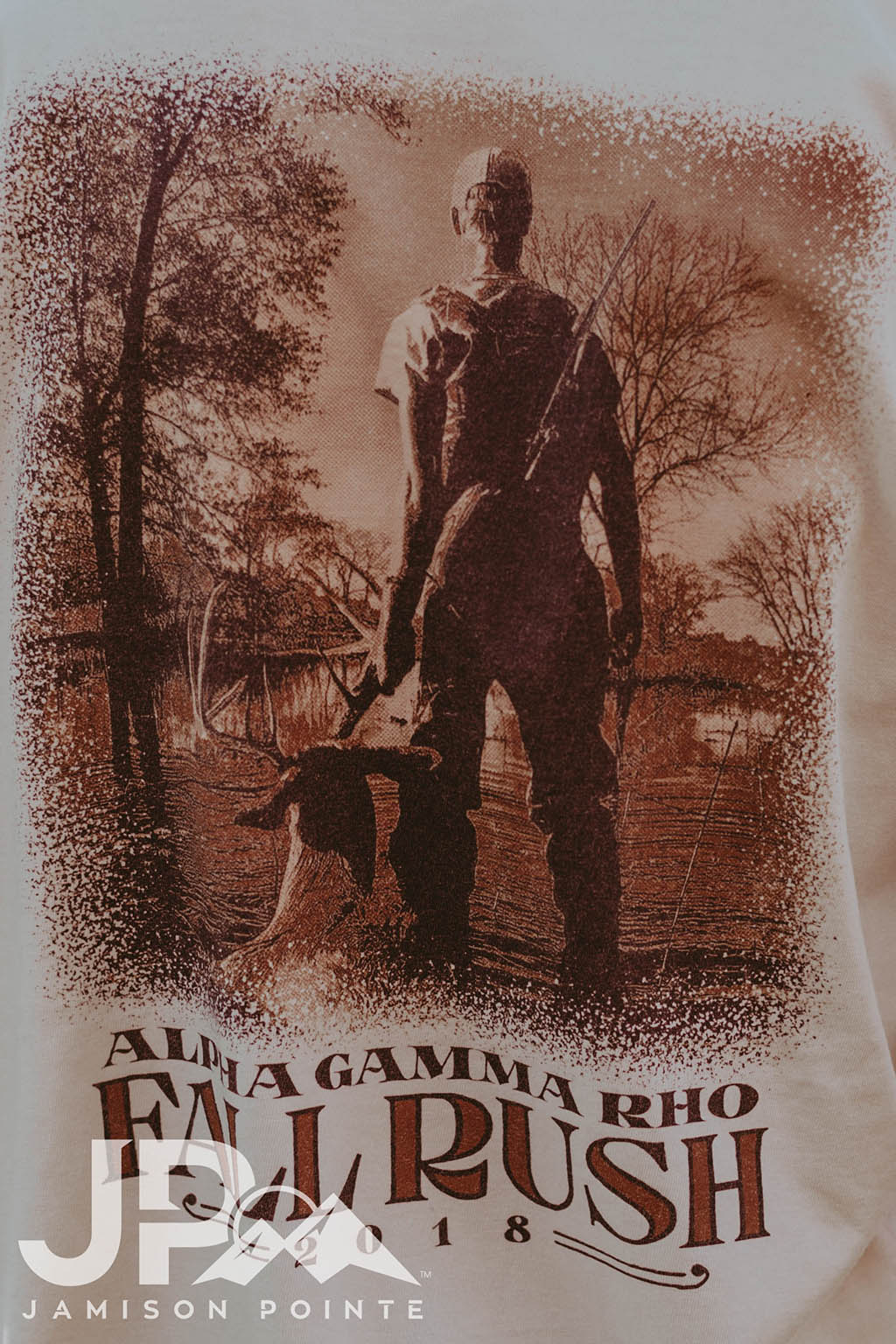This sepia-toned, vertical poster advertises the Alpha Gamma Rho Fall Rush event in 2018. The main text, "Alpha Gamma Rho," is prominently displayed in bold, all-capital red letters with "Fall Rush" beneath it. Below that, "2018" appears in white letters. In the lower left corner, there's a watermark featuring the letters "JP" with a small mountaintop and the words "Jameson Point." The illustration portrays the back of a male hunter standing by a body of water surrounded by trees. He is dressed in overalls and a hat, with a shotgun or rifle secured in his backpack. The hunter holds the antlers of a deceased deer with his left hand. The edges of the poster are feathered out on a white background, adding to its rustic aesthetic.